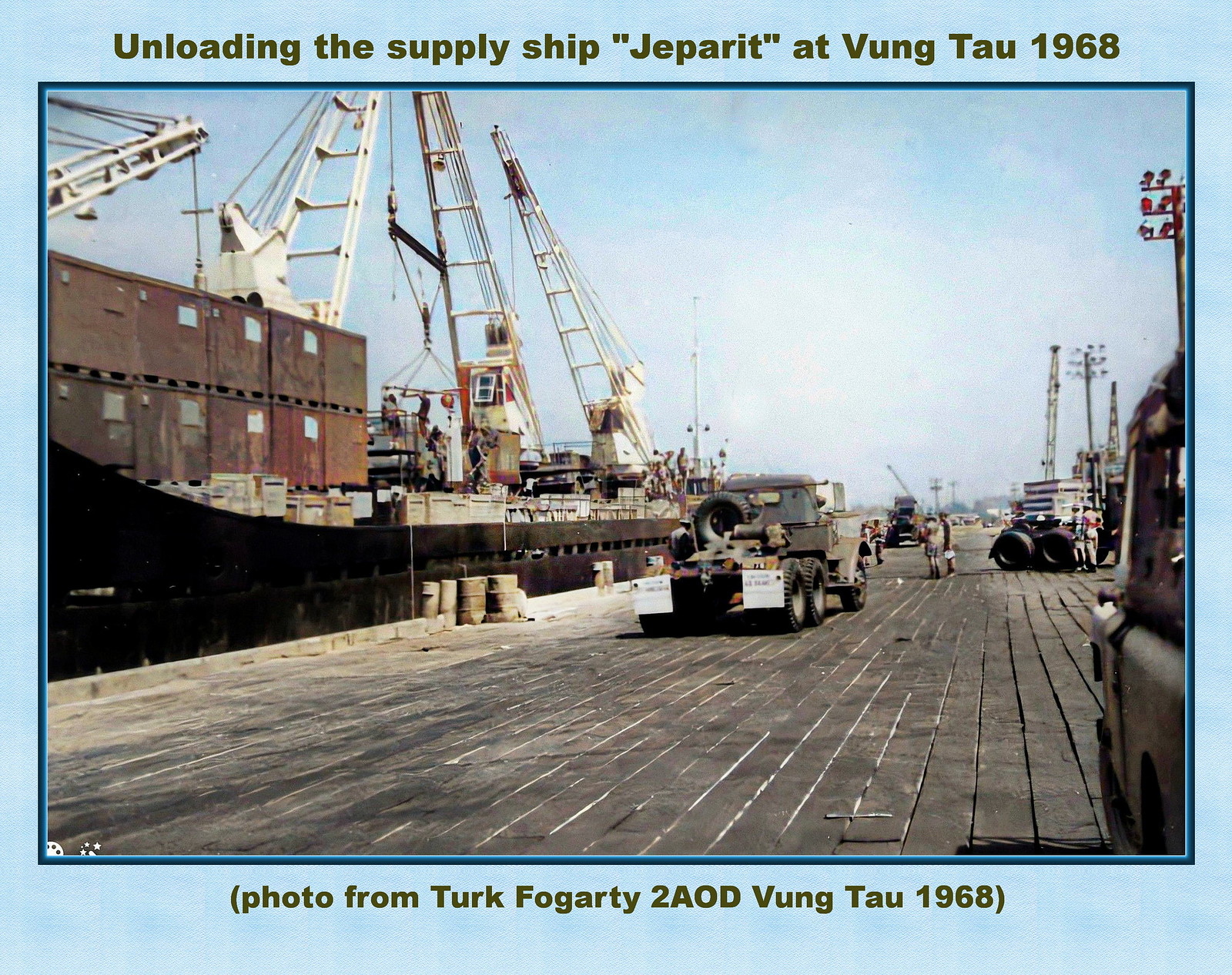This detailed image captures a bustling harbor scene from 1968 in Vung Tau, Vietnam, with a light blue border framing the photograph. The top of the image features the caption: "Unloading the supply ship Jeparit at Vung Tau, 1968." In the foreground, a military vehicle drives across a large wooden dock lined with numerous barrels and supply containers, many of which are brown and rusted. Cranes towering over the dock are in the process of unloading the supply ship Jeparit, which is moored nearby. The sky above is a vivid blue, dotted with white clouds, enhancing the historical and military setting of this vibrant, full-color photograph. Several people can be seen working amidst the cargo, adding to the sense of activity and urgency. The bottom of the image bears the text: "Photo from Turk Fogarty to AOD Vung Tau, 1968," further authenticating its historical significance.